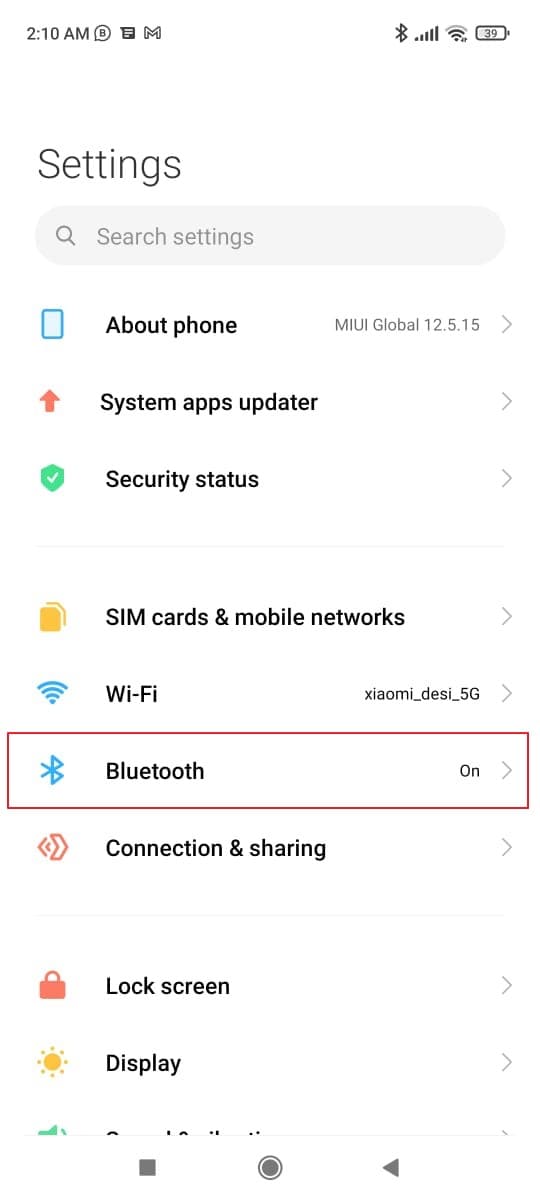A detailed screenshot of the settings section of a mobile phone is displayed. At the top left, the word "Settings" is prominently featured. Directly below it, a search bar labeled "Search settings" is available for user convenience. The settings menu is organized into a list, with each entry accompanied by an icon on its left side. Starting from the top, the entries are as follows:

1. "About phone" with a sub-label indicating "MIUI Global 12.5.15." 
2. "System app updater." 
3. "Security status." 
4. "SIM cards & mobile networks."
5. "Wi-Fi," which shows an active connection to "Xiaomi_Desi_5G" on the right.
6. "Bluetooth," which is turned on and distinctly highlighted by a red box.

Further down the list are additional entries:
7. "Connection & sharing."
8. "Lock screen."
9. "Display."

Each row has an arrow pointing to the right, indicating further options or sub-menus available upon tapping. 

In the status bar at the top of the screen, several icons are visible:
- A timer displaying "2:10" in the top left corner.
- A Google Mail icon just to the right of the timer.
- A battery icon showing a 39% charge level.
- A Bluetooth icon, confirming its active status.

The detailed elements and organization of this settings menu provide a user-friendly interface for managing various aspects of the phone.